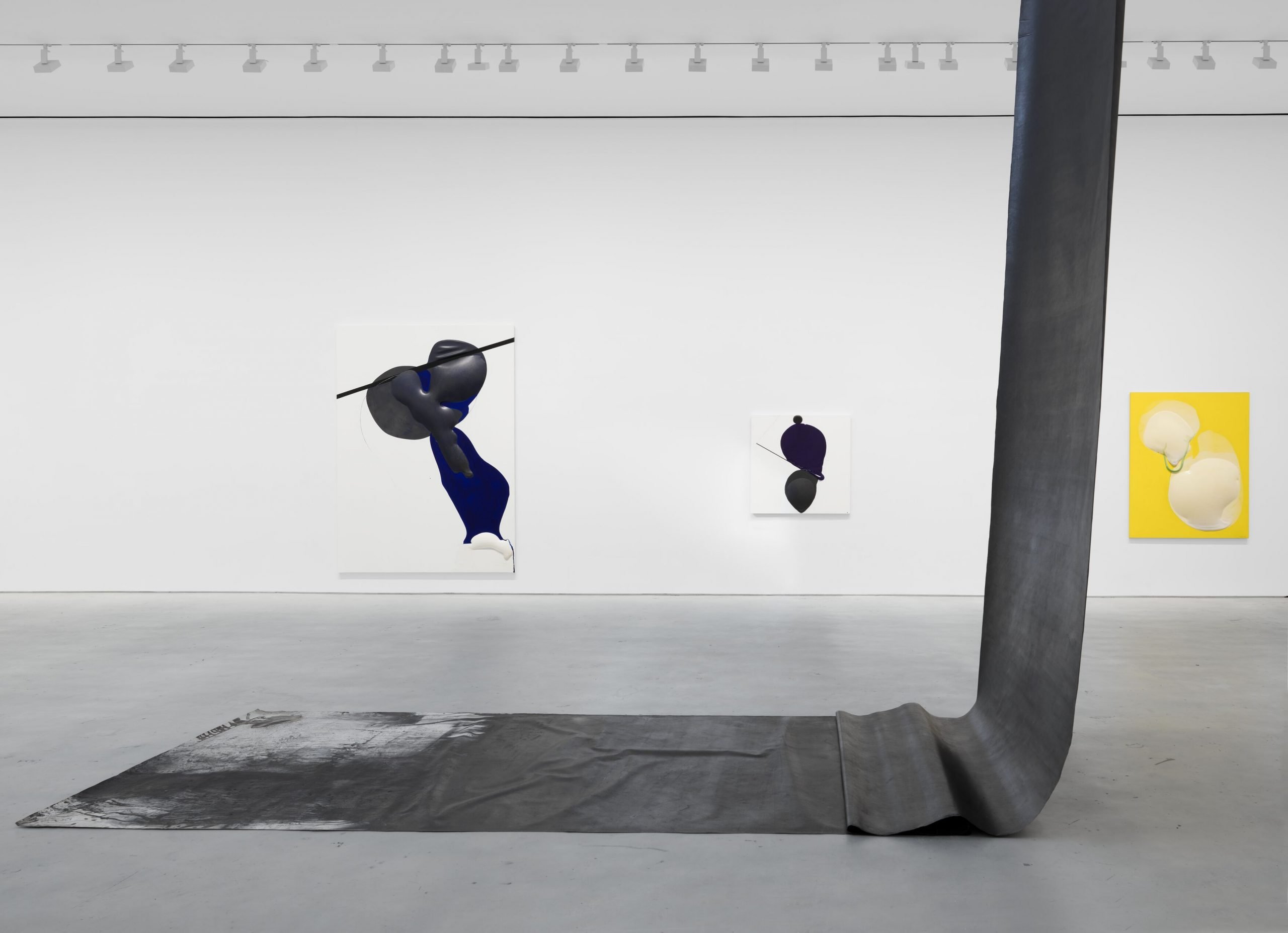The photograph captures the interior of a spacious art gallery with bare white walls and a gray concrete floor, featuring a high ceiling lined with track lighting. Dominating the foreground is a wide piece of black fabric, gracefully draping from the unseen ceiling and pooling onto the floor, resembling a long runner or rug. In the background, the stark white wall hosts three abstract canvases of varying sizes. The leftmost canvas is a large black-and-white piece, followed by a smaller black-and-white square canvas in the center. The rightmost canvas stands out in bright yellow, featuring a distinctive 3D plastered arc. The room's minimalistic design and the contrasting colors of the artworks create a striking visual composition.